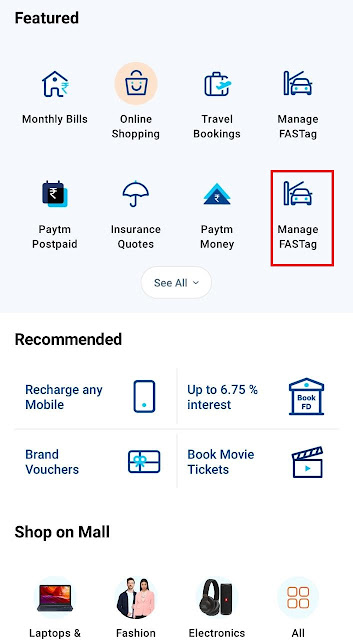This is a screenshot from a mobile application, likely Paytm, a digital wallet services platform in India, similar to PayPal. The interface is divided into two sections: "Featured" and "Recommended." 

In the "Featured" section, users can access monthly bills, online shopping, travel bookings, manage FASTag, Paytm Postpaid, insurance quotes, and Paytm Money. There is also an option to see all items in this category.

The "Recommended" section offers quick access to recharge any mobile, brand vouchers, up to 6.75% interest savings, and booking movie tickets.

At the bottom, there is another category labeled either "Shop on Mall" or "Shop on Mail" (partially cut off), featuring items in four categories: laptops (partially cut off), fashion, electronics, and an all-encompassing option to see all available categories.